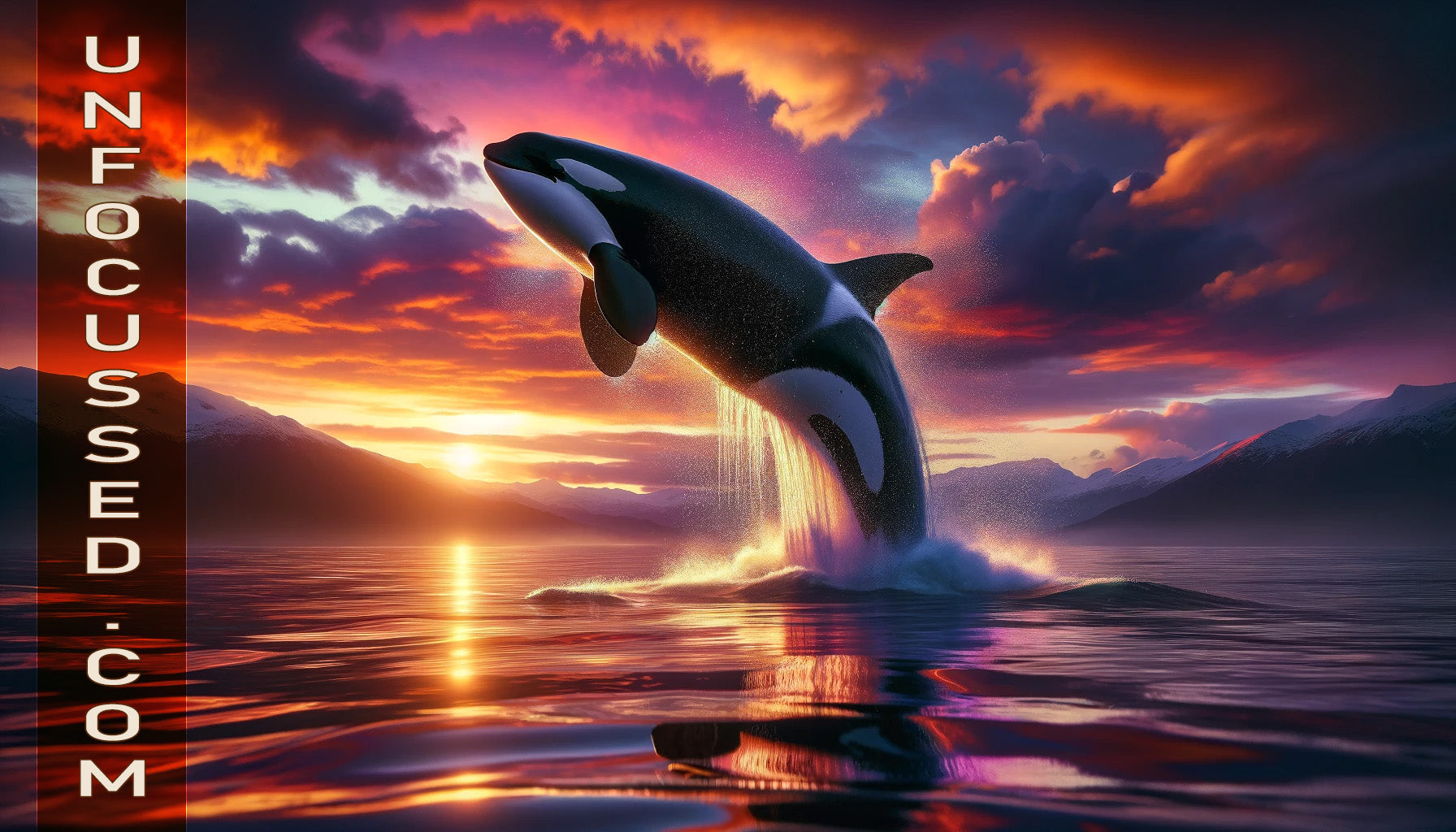This digital image strikingly resembles a photograph but is unmistakably artificial. It captures a majestic killer whale, or orca, completely airborne with only its tail still touching the calm water. The water is serene except for the splashes created by the whale's leap. Surrounding its tail are white waves, adding contrast to the scene. In the background, towering mountains frame the horizon with the sun either setting or rising, casting a stunning array of pink, purple, red, and yellow hues across the sky and reflected in the water. These vibrant colors imbue the entire image with a surreal, almost dreamlike quality. The majestic quality of the orca is further emphasized by the cloudy sky, which is painted with the dramatic reds and oranges of the setting sun. On the left side of the image, the vertical, white text "unfocused.com" subtly suggests a potential use as a digitally crafted wallpaper.